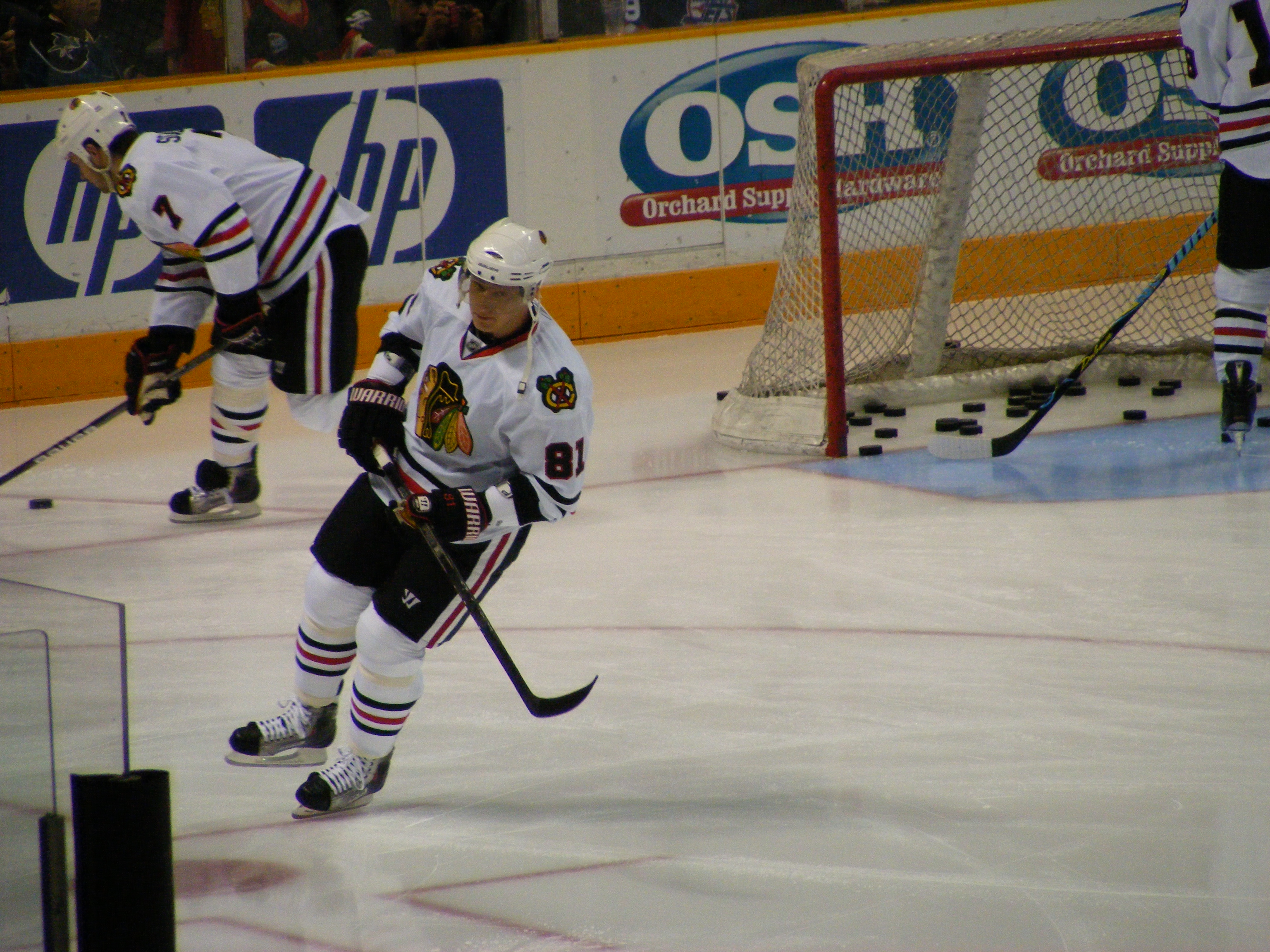This detailed photograph captures a practice session of a professional ice hockey team. The central focus is on three players in white jerseys with a Native American head logo and black shorts; numbers 81 and 7 are visible. They are on an ice rink featuring red and blue markings and are actively engaged in the practice, maneuvering their black hockey sticks to control the puck. One player, leaning heavily to his right, is seen preparing for a move. The goal in the far right is framed with a red border and white net, filled with numerous pucks from the warm-up session. The ice surface is pristine white with distinct red stripes. Behind the rink, a glass barrier capped with prominent yellow and white trim separates the players from spectators. The ice rink's sponsors, HP and Orchard Supply Hardware (OSH), are prominently displayed in the background, adding a commercial touch to the practice scene.